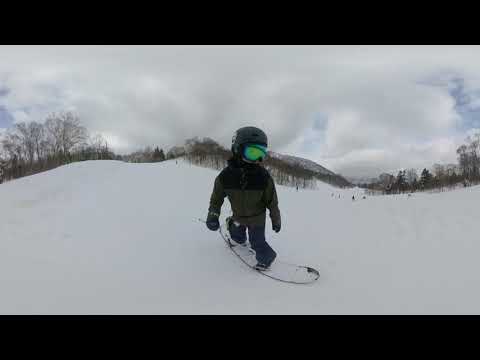This digital photograph captures a person actively snowboarding in a snow-covered landscape. Dressed in a coordinated snowsuit, the snowboarding enthusiast sports blue pants and a striking black and dark hunter green jacket. Their essential accessories include a dark helmet and reflective bluish-green goggles that stand out vividly. The snowboard beneath them is visibly sprinkled with snow, highlighting the action amidst the wintry scene. The backdrop of the image features a mostly overcast sky with thick white clouds, allowing only hints of blue to peek through. Along the horizon, bare trees with no leaves frame the snowy setting, adding to the desolate beauty of the environment. There are no other people immediately surrounding the snowboarder, although several individuals can be spotted further downhill. The overall color palette of the image includes various shades of green, yellow, black, blue, and white, enhancing the visual depth of this outdoor adventure.